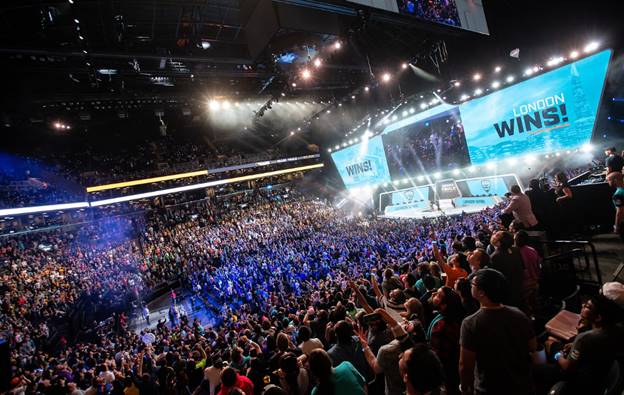This image captures a bustling indoor arena filled to capacity with an excited audience. Dominating the scene is a white stage at the front, illuminated by bright blue lights and overhead spotlights. The stage features three men who appear to be wrestlers, engaging the crowd. Prominently displayed on a large screen to the right is the message "LONDON WINS!" in vibrant, capital letters. Despite the darkness that shrouds much of the arena, glimpses of audience members' clothing in blacks, light blues, tans, and yellows can be seen, with many attendees holding up their phones to film the event. High above, a metal frame and additional screens enhance the lively atmosphere of this competition, as the audience cheers with hands raised, adding to the dynamic energy of the scene.